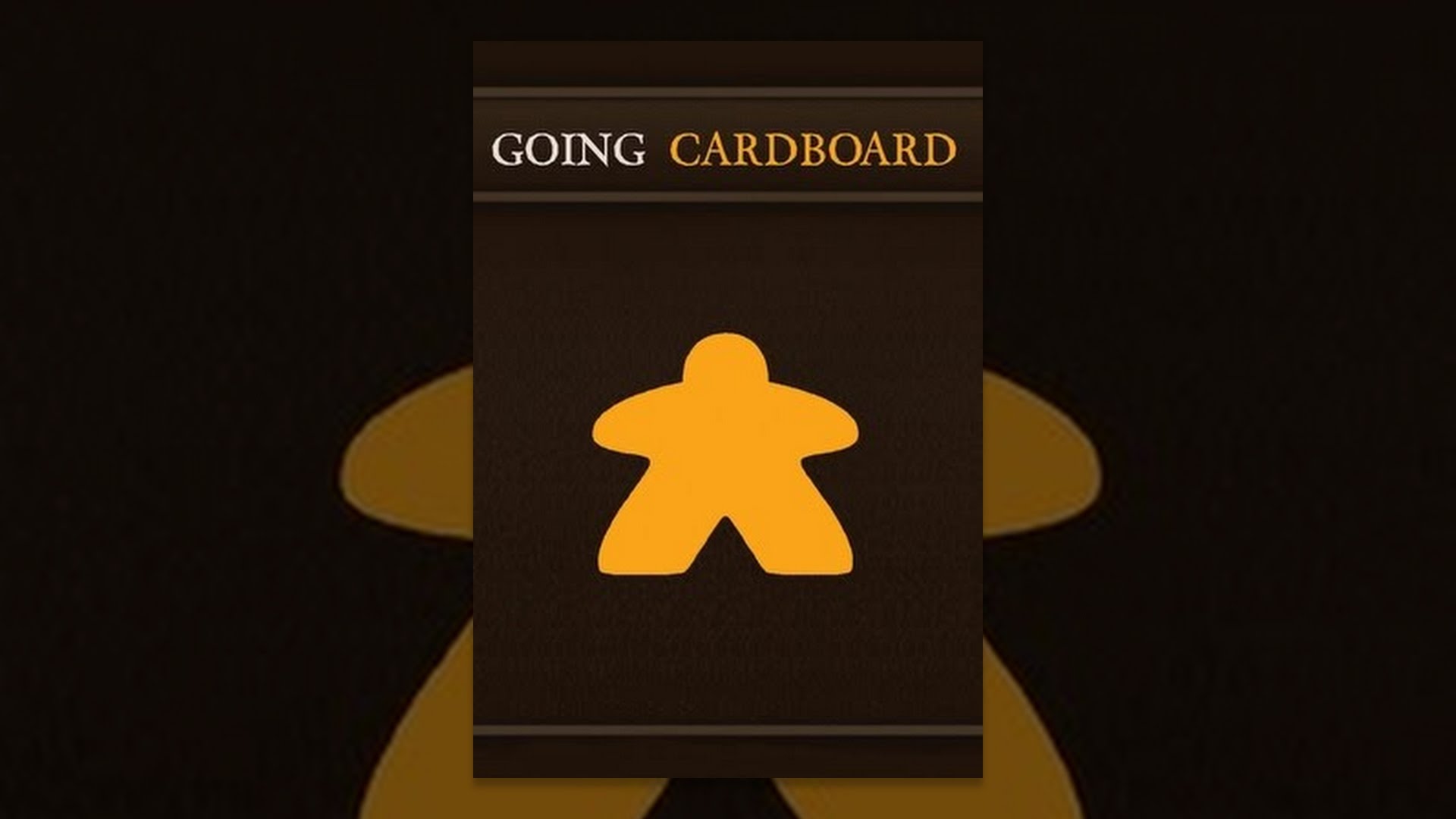The image showcases a visually striking logo. At its center is a vertically-oriented, brown rectangular area with the phrase "GOING CARDBOARD" displayed in all capital letters. The word "GOING" is written in white, while "CARDBOARD" is in yellow. This text is framed by thin, light brown lines along the top and bottom of the rectangle. Within this central rectangle, there is a simple, abstract outline of a gingerbread-man-like figure in yellow. The background is a flat, dark black, upon which fragments of the same gingerbread-man-like figure, rendered in yellow, are repeated, creating a mise en abyme effect. This intricate layering evokes depth and complexity, making it unclear whether the brown rectangle is physically resting on a surface or digitally superimposed. The minimalist design lacks facial features on the abstract human outlines, enhancing the modern, streamlined aesthetic.